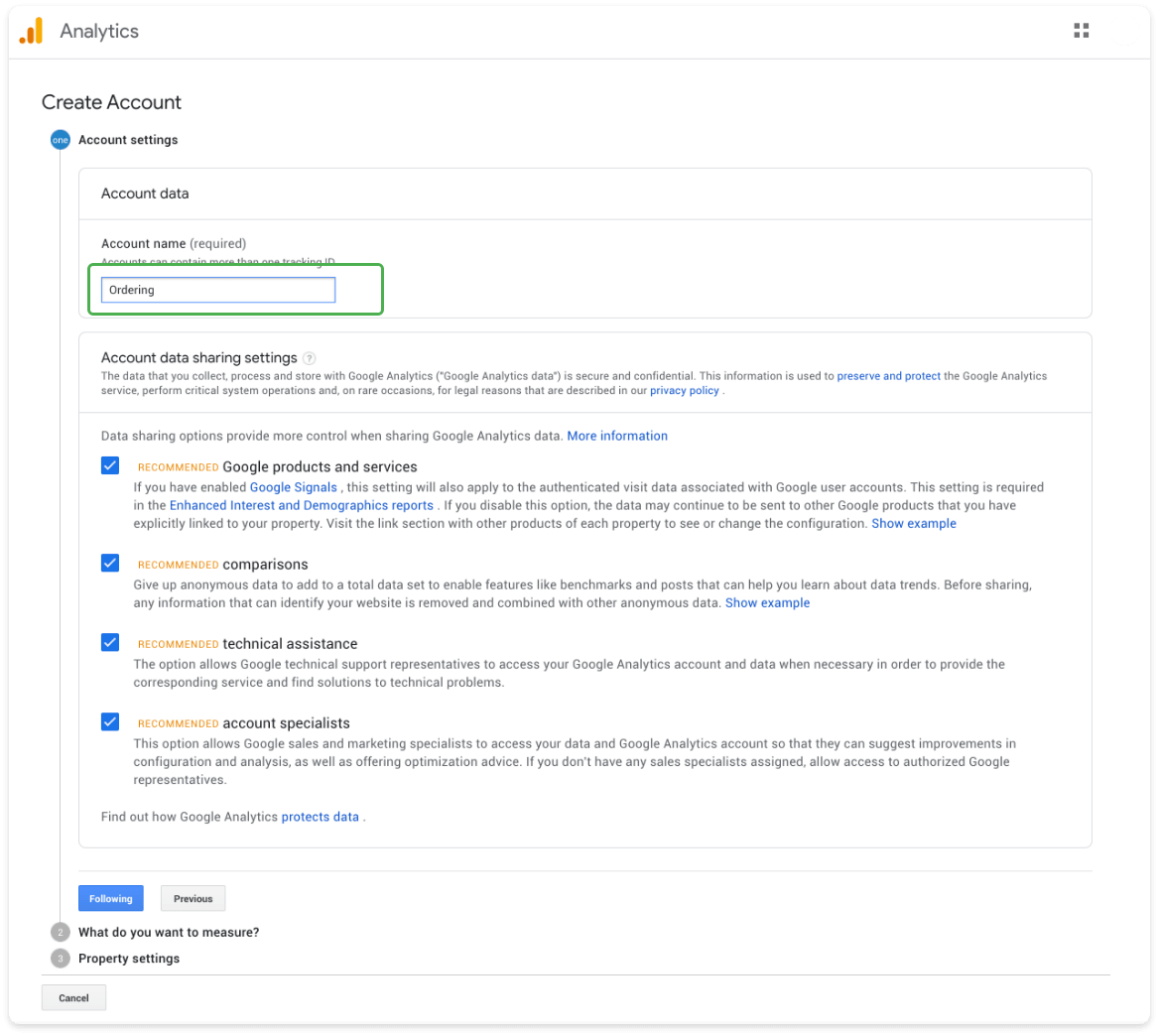The image is a detailed schematic created for analytical purposes. At the top, there is a bar graph with vibrant orange and yellow hues, accompanied by the word "Analytics" prominently displayed in print. Moving to the right, four simple squares come together to form a gray cube. Below this, a faint gray line marks the transition to the next segment, labeled "Create Account."

Under this title, there is a circle containing the numeral "1" and the text "Account Settings." Progressing downward, the section is labeled "Account Data," followed by "Account Name," which is marked as "Required." A green box encloses a blue box that reads "Ordering." 

Further down, the "Account Data Sharing Settings" section features four checked areas, each with the word "Recommended" in orange text. Below this, a blue box labeled "Following" can be checked, along with a gray box marked "Previous." 

Continuing downward, a circle containing the number "2" asks, "What do you want to measure?" Next, a gray circle with the number "3" denotes the "Property Settings" section. Another faint gray line runs across the design, and in the bottom left-hand corner, there is a gray box labeled "Cancel."